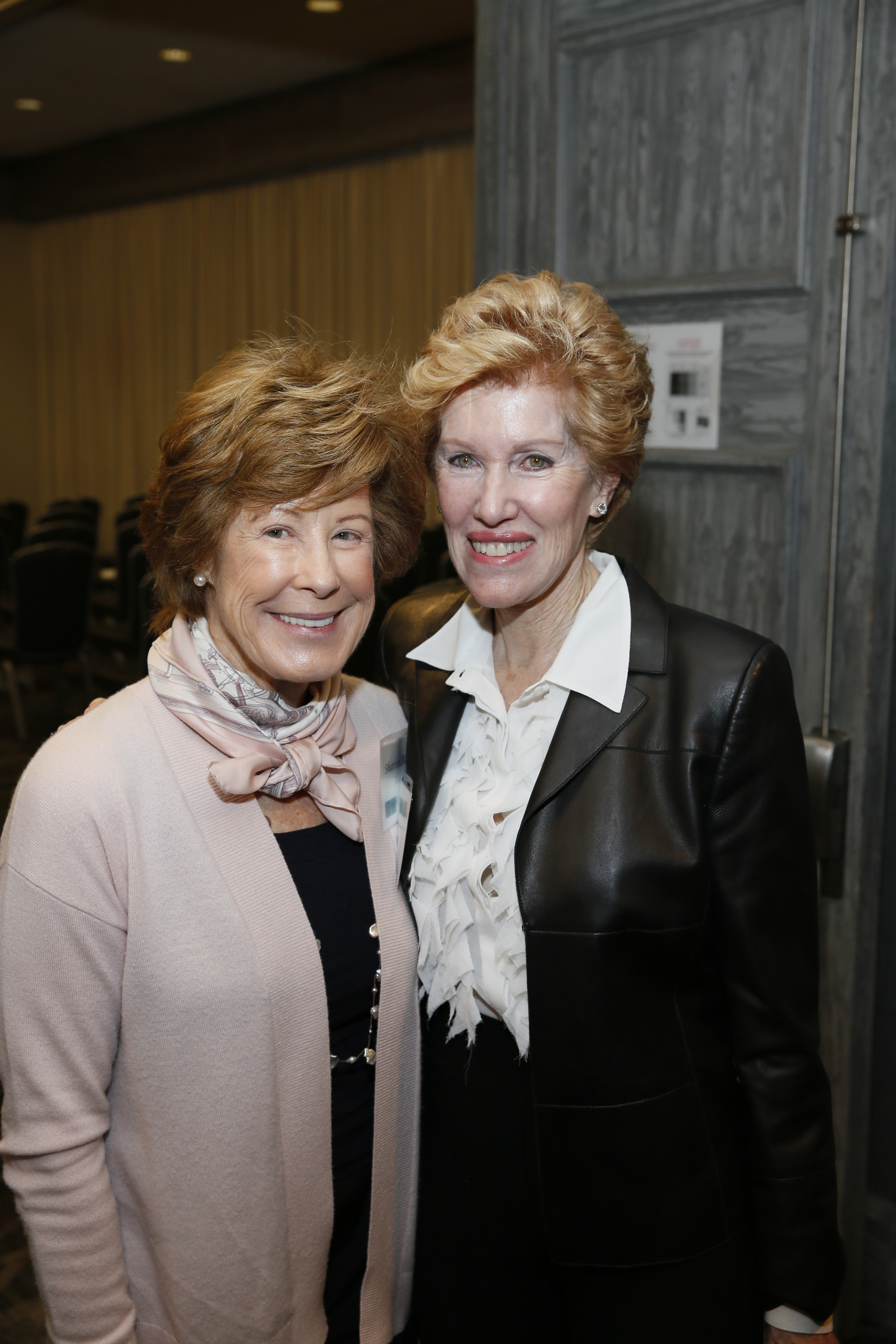The image features two older women centered in the frame, both smiling warmly at the camera. The woman on the left has medium-length, brownish-reddish hair and is dressed in a pale pink sweater cardigan over a black top. She also wears a pink scarf around her neck, and possibly a second scarf with a white and black pattern, along with a long necklace and pearl earrings. Next to her, on the right, is a woman with a similar hairstyle but in a lighter blonde shade. She wears a black leather jacket over a white, collared shirt with frilly or ruffled detailing. Both women are holding their hands and arms down next to their bodies. The background includes a gray door to the right and a light brown wooden wall to the left, potentially indicating that they are in a conference room with visible chairs and curtains. They appear to be in their late 60s to early 80s.